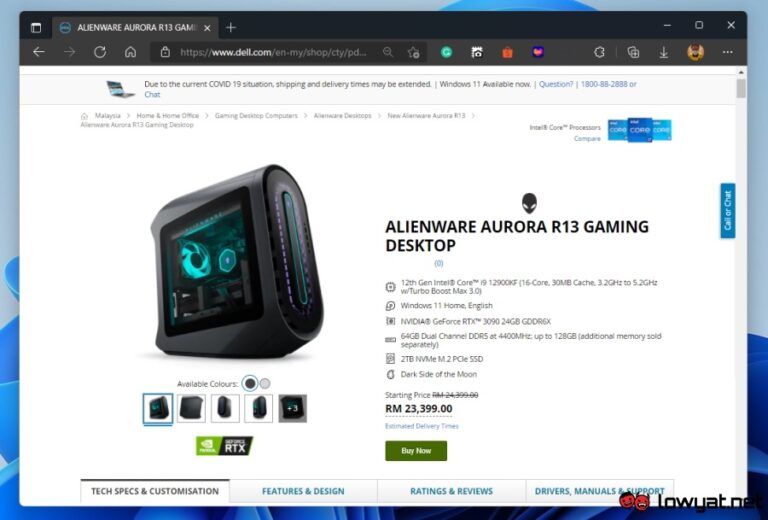The image showcases a website featuring a detailed product page for the Alien Aurora R13 Gaming Desktop. Surrounding the main content is a decorative blue border, with a darker blue design encircling it. At the top of the page, the background is black and displays an open browser tab titled "Alien Aurora R13 Game."

The browser interface is visible and includes a left arrow, right arrow, refresh button, and web address in the address bar, accompanied by several icons on the right side. The main content area of the webpage is white and contains a notice about potential shipping and delivery delays due to the COVID-19 situation. It also includes promotional text indicating that Windows 11 is now available, along with a phone number and chat option for customer inquiries.

Further down, the image of the product is prominently displayed in two available colors: black (selected) and gray. Five additional images showcase the Alien Aurora R13 Gaming Desktop from different angles. The product description, written in bold, capital letters, reads "ALIEN AURORA R13 GAMING DESKTOP." Pricing information is listed as "R $2,399" (or a similar format with specific currency details). The page includes a call-to-action "BUY NOW" button with a green background.